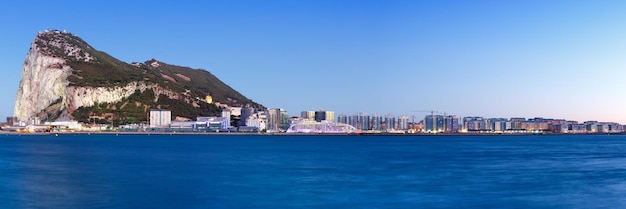A wide panoramic photograph captures a coastal cityscape with a dramatic mountain and expansive ocean. The image transitions from a clear blue sky, which fades from dark blue at the top left to a lighter blue towards the lower right, to a deep, dark blue ocean that occupies the first 30-40% of the view. On the left-hand side, a towering mountain rises sharply, occupying about half of the vertical space. The mountain's left face is predominantly white granite, with the right face covered in green vegetation atop light brown earth.

Nestled at the base and extending toward the right of the mountain is a sprawling cityscape with skyscrapers and high-rise buildings, though they appear small due to the photograph's distant vantage point. The buildings, despite being large, only take up about 10% of the image's height and are outlined against the ocean. Among the various structures, colorful shipping containers indicate an industrial or port area on the right side of the image.

The overall palette is dominated by blues from the sky and ocean, with the mountain adding contrasting hues of green and brown. The image suggests a bustling urban area with ongoing construction, evidenced by cranes amongst the high-rises, framed by natural beauty and dominated by the imposing mountain feature.